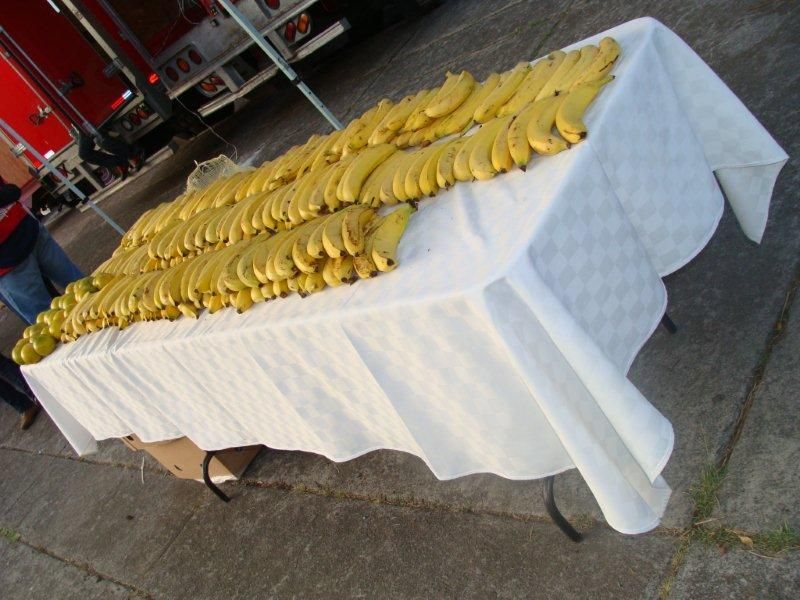The photo features an angled perspective of a long folding table covered with a white checkered tablecloth. The checkered pattern consists of varying shades of white and gray, and the cloth appears wrinkled in certain areas. The table is set on a concrete floor interspersed with patches of grass. Placed across the table are three rows of bananas, with many of them stacked on top of each other, especially on the left and towards the end of the table. Some parts of the middle and near end rows have fewer bananas, exposing a single layer and an open space at the bottom right where bananas have already been taken. On the far left corner of the table, there's a pile of mangoes, roughly around 20 in number. Additionally, there’s a box positioned underneath the table on the bottom left. In the background, semi-truck trailers are partially visible, along with a glimpse of a man dressed in blue jeans and a blue shirt. The legs of the table can be seen touching the concrete ground. Overall, the scene suggests a market or a serving setup, accentuated by the abundance of fruits and the utilitarian surroundings.